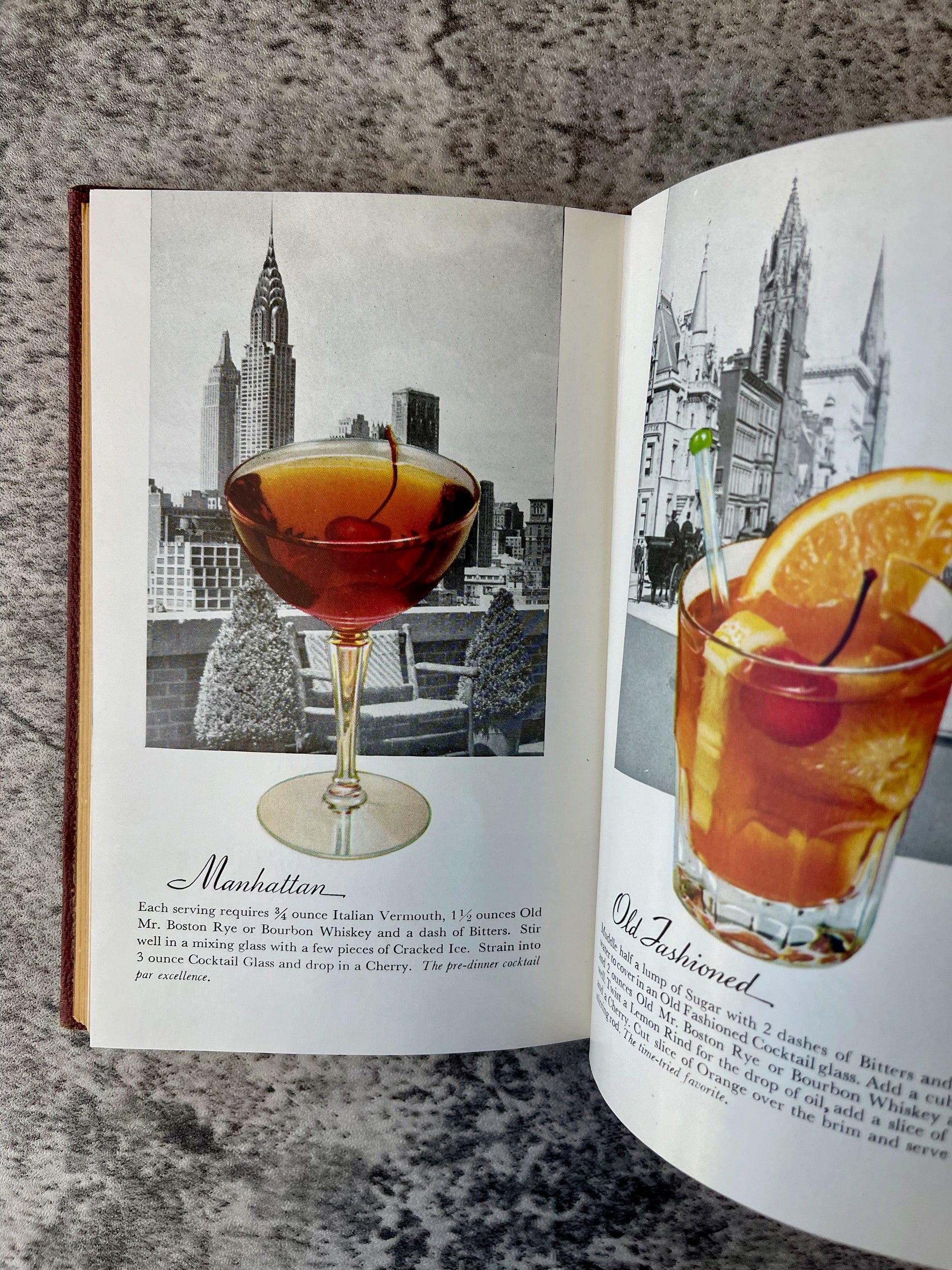This captivating image showcases an open book focusing on classic cocktails amidst urban settings. On the left page, the spotlight is on a Manhattan, depicted as a brownish-orange drink served in a martini glass with a cherry. The background features a black and white image of a cityscape with tall skyscrapers, adding a touch of sophistication. The detailed text describes the recipe, calling for ¾ oz Italian vermouth, 1½ oz old mixture Boston rye or bourbon whiskey, and a dash of bitters, stirred with cracked ice and strained into a 3 oz cocktail glass, crowned with a cherry as the pre-dinner cocktail par excellence.

On the right page, another enticing cocktail, the Old Fashioned, is presented. This drink is shown in a different type of glass with an orange liquid containing a cherry and orange slices. The background continues the urban theme with a black and white image of an old-fashioned city scene. Below this image, the text provides a description of the cocktail, maintaining the book's purpose of educating readers about mixed drinks. The clarity and brightness of the image suggest it was taken under natural lighting, enhancing the visual appeal of the detailed illustrations and background cityscapes.